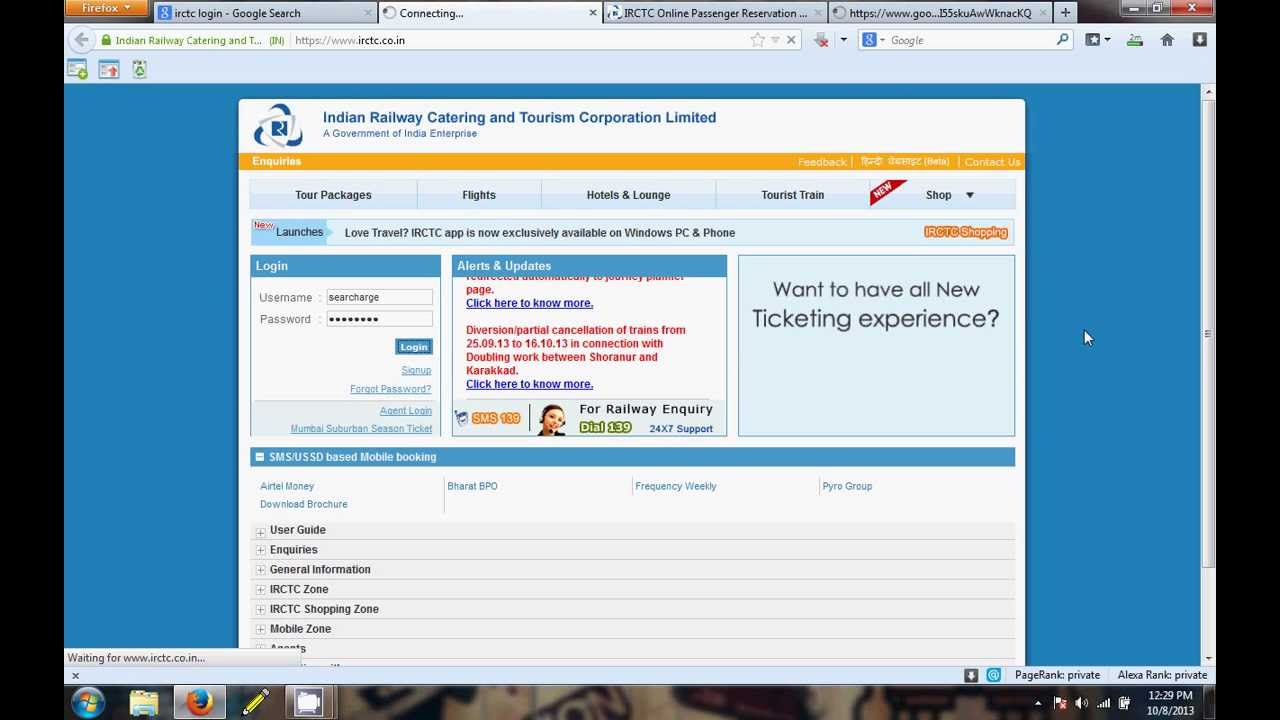In this detailed screenshot of a computer screen, we can discern that the user is running Windows 7, as indicated by the familiar Windows icon located in the lower-left corner. The taskbar at the bottom reveals several icons, including one for Firefox, suggesting that this is the primary web browser being used. Additionally, the time displayed is 12:29 PM, and the date reads October 8, 2013.

The main screen showcases an open web browser window navigated to the URL www.irctc.co.in, the official website for the Indian Railway Catering and Tourism Corporation Limited (IRCTC). At the top of the browser, multiple tabs are open, with the currently active tab focused on the IRCTC site.

Prominently displayed at the top of the webpage is the IRCTC's full name, "Indian Railway Catering and Tourism Corporation Limited," followed by a yellow banner labeled "inquiries." Various clickable sections are organized on the site, including "Tour Packages," "Flights," "Hotels and Lounge," "Tourist Train," "Shop," "Launches," and "Love Travel." A notable banner advertises the availability of the IRCTC app exclusively for Windows PCs and phones.

The website features a login section where users can enter their username and password. Additionally, there are alert and update notifications. A highlighted segment invites users to "Want to have all new ticketing experience," preceded by brief introductions to several zones like the "User Guide," "Inquiries," "General Information," "IRCTC Zone," "IRCTC Shopping Zone," and "Mobile Zone."

The page's color theme primarily uses blue and white tones, with occasional accents of yellow and red text, giving it a clean and organized aesthetic.